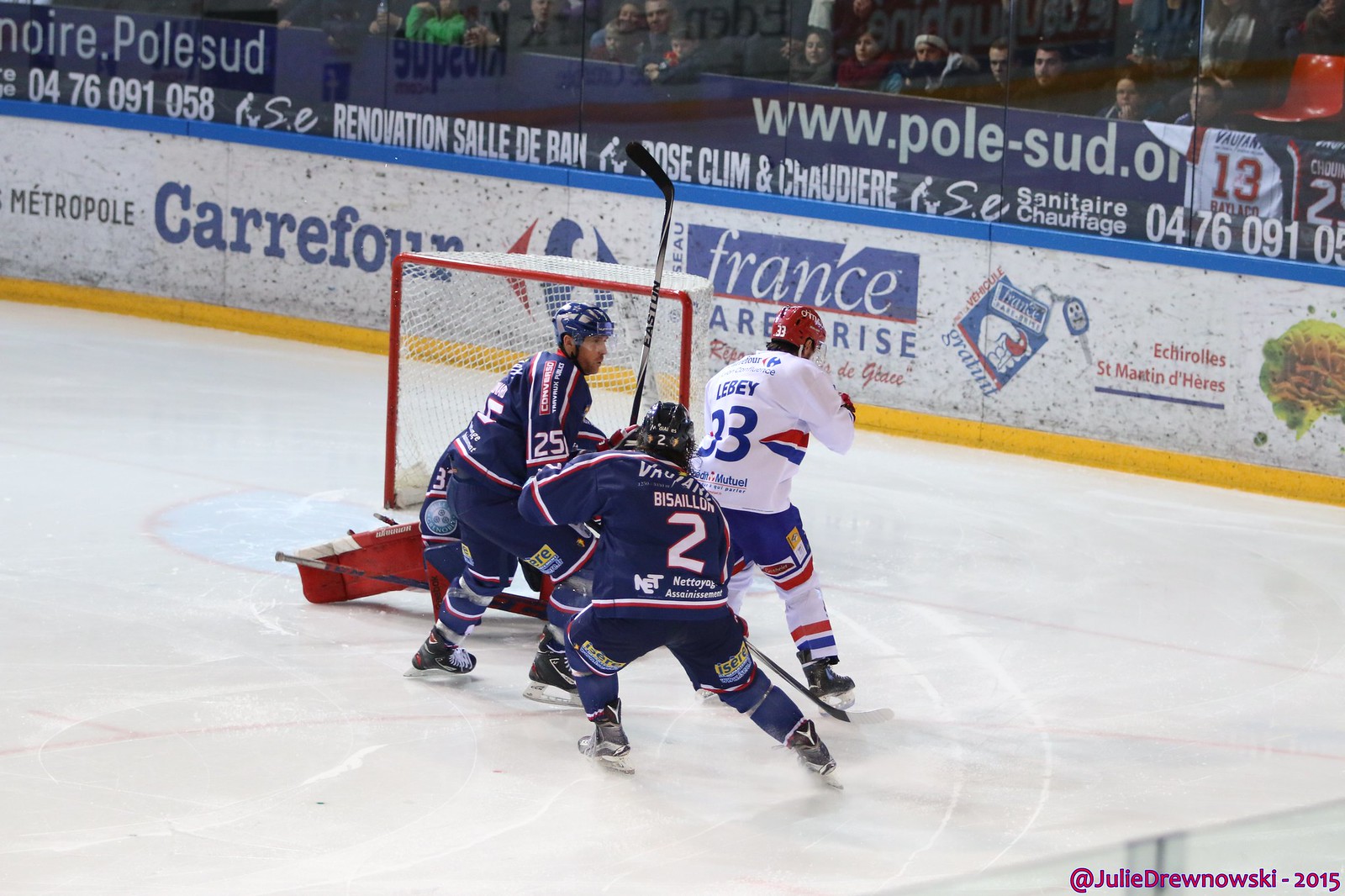The image captures an intense moment in a hockey game featuring three players. The players include one in a white jersey with the number 33 and two in navy blue jerseys with the numbers 25 and 2. They are all vying for control near the goal. The player in the white jersey is not holding his stick visibly, while the player closest to the goal, who has his face partly visible, is holding his stick in the air. The other blue-jerseyed player has his stick down on the ice. Behind them, the boards display various sponsorships, including phrases like "care for France," "France are to rise," "Archioli St. Martin D. Harris," and "www.pole-sud.org," alongside an image of car keys. The background further reveals a crowd of spectators dressed in warm clothing, seated in red chairs behind plastic shielding, intently watching the action unfold on the ice.